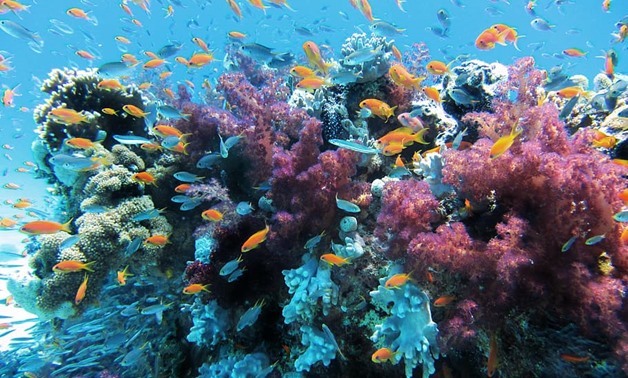The image captures a vibrant and lively underwater scene centered around a healthy coral reef. The water is a deep, uniform blue, and exceptionally clear, with the coral displaying an array of bright, captivating colors including aqua blue, dark purple, dark green, light green, creamy whites, and notably, a striking pinkish-purple coral in the middle with delicate, hair-like filaments flapping in the water. Surrounding this vibrant coral reef are hundreds of small to medium-sized fish, predominantly in solid orange and blue hues, creating a dynamic, swirling pattern as they swim through the scene. To the left of the image, there are distinctive patches of white coral and some prominently bright purple coral, enhancing the rich tapestry of colors. The overall scene is one of an abundant, thriving marine ecosystem teeming with life and color.